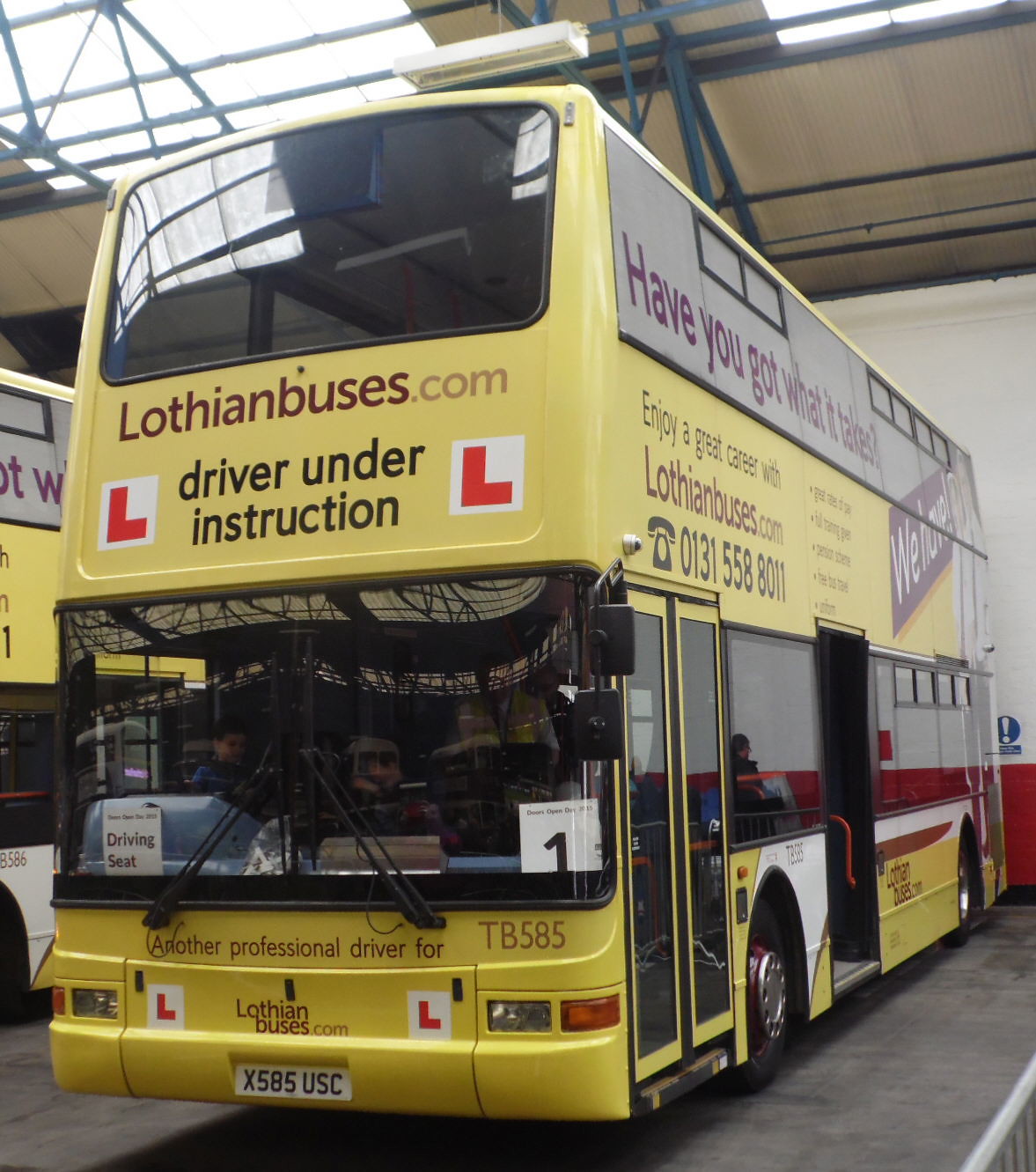A striking double-decker bus, predominantly painted in vibrant yellow, occupies the central focus of the image, taking up nearly the entire frame. The bus is parked in a bus depot, against a background wall painted in white and red. Eye-catching text on the bus’s side promotes a career with Lothian Buses, stating, "Enjoy a great career with LothianBuses.com," and challenging potential recruits with, "Have you got what it takes?" Additional signage reads, "Welcome," "Driver under instruction," and "Another professional driver for Lothian Buses." The bus's black tinted windows, license plate X585 USC, and a mix of black, yellow, red, white, blue, and maroon lettering add to the visual complexity. Upon closer inspection through the windows, one can glimpse the silhouettes of passengers inside, and there's a noticeable glare, possibly suggesting a figure standing nearby. The vehicle is positioned in a marked parking slot within the depot, under a light gray top panel and set against a grounded, reflective surface.